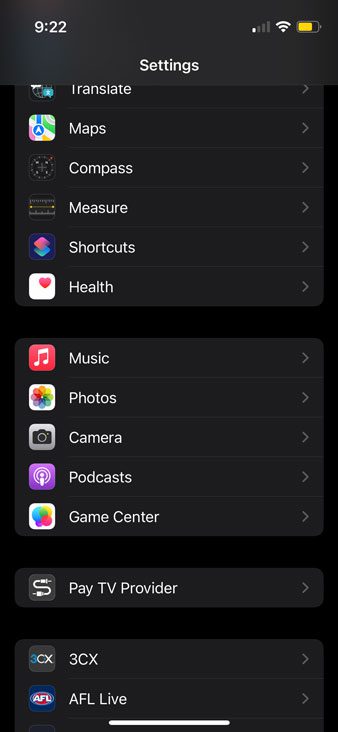The image displays a detailed screenshot of the settings menu on a cell phone. At the top of the screen, typical status indicators are visible: a clock in the top left corner, a battery meter in the top right, and a Wi-Fi signal icon. The settings header is prominently displayed in white text against a black background. 

Below this heading, an array of menu buttons is presented, each accompanied by icons on the left side. These menu options include:

- **Translate**: Represented by its corresponding icon.
- **Maps**: With a map pin icon.
- **Compass**: Displayed with a compass icon.
- **Measure**: Featuring a ruler icon.
- **Shortcuts**: Marked by a shortcut icon.
- **Health**: Indicated with a heart or health-related icon.
- **Music**: Accompanied by a music note icon.
- **Photos**: With a camera or photo icon.
- **Camera**: Identified by a camera icon.
- **Podcast**: Represented by a microphone or podcast icon.
- **Game Center**: Featuring a game controller icon.
- **Pay TV Provider**: Displayed with a TV icon.
- **3CX**: Accompanied by an appropriate icon, likely related to communication.
- **AFL Live**: Marked by an icon relevant to sports or AFL.

All these menu options are situated against a sleek black background, providing a clear and organized layout for easy navigation.